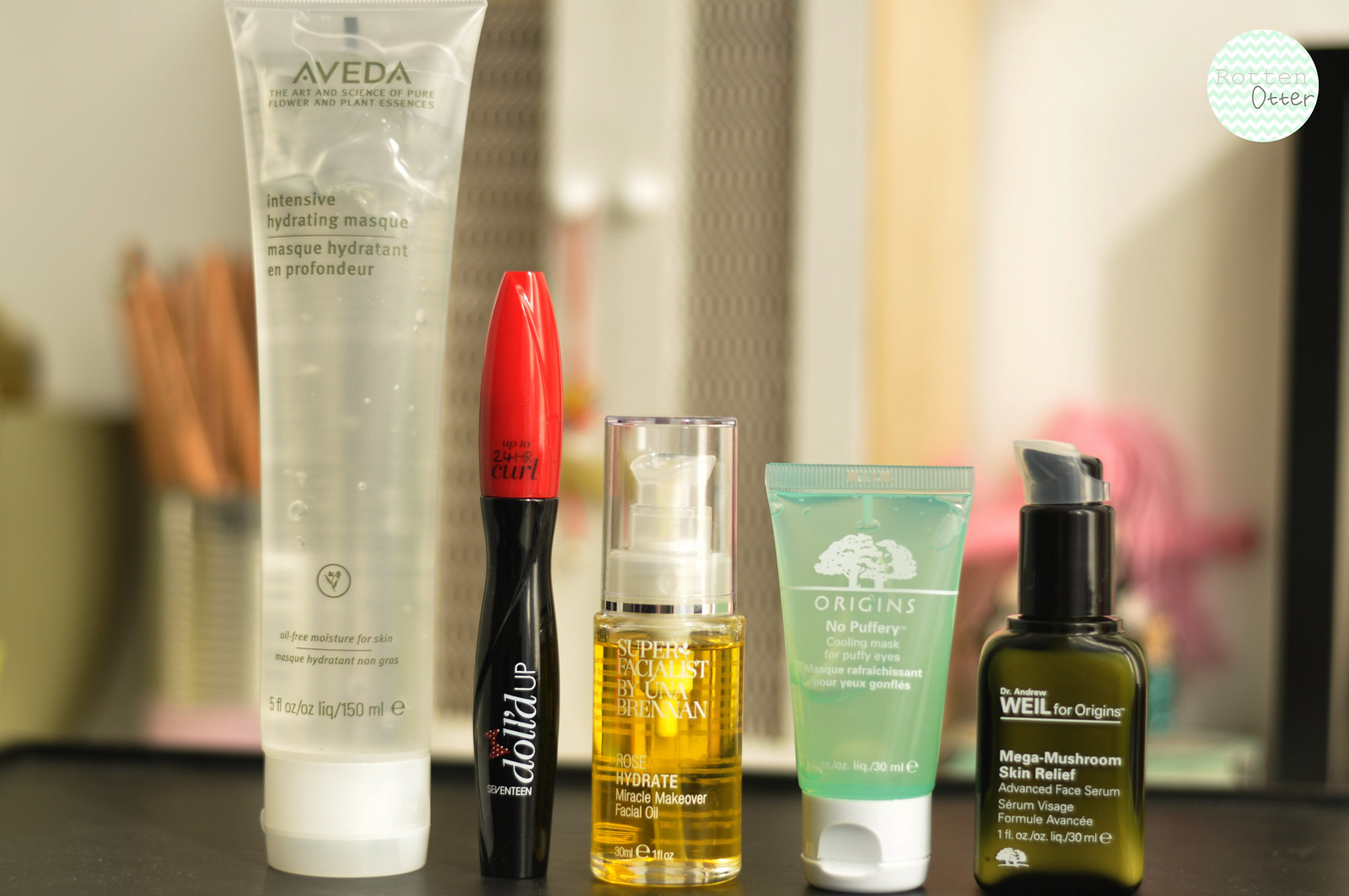The photograph showcases an array of sophisticated skincare and makeup products displayed meticulously on a dark wooden surface. The background of the image is artfully blurred to ensure the products remain the focal point, though a keen eye might notice the faint outline of a mug or pot, perhaps housing a cactus, alongside a jar and what appear to be cabinet door handles, suggestive of a bathroom setting.

In the foreground, the first item featured is a large, transparent tube with a white lid, containing a clear, gel-like substance from Aveda. Adjacent to this is a sleek, black tube resembling a mascara container, capped with a striking red lid, emblazoned with the phrase “dolled up” in white text. 

Next in line is a distinctive pump-action container, characterized by its transparent body holding a sunshine yellow liquid, coupled with a clear lid and a white pump labeled “hydrate,” though the remaining text is not fully visible. 

Following this is a smaller, frosted, see-through tube containing a pale green product and topped with a white lid, identifiable as an offering from Origins. 

Completing the collection is an olive green, dark glass bottle equipped with a black and gray pump lid, inscribed with “Wheel for Originals” or possibly "Origins."

Each product is thoughtfully positioned to highlight its unique design and purpose, making the arrangement both visually appealing and informative.